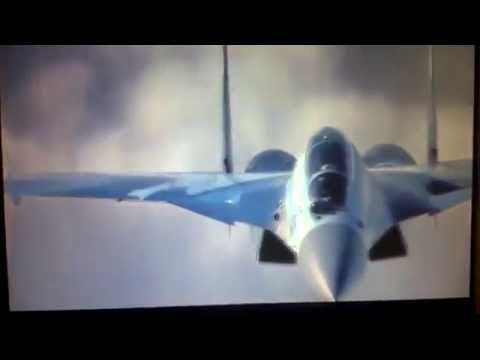The image captures a head-on view of an incoming fighter jet, depicted photographically as part of another screen display. The image quality is notably poor, characterized by blurriness and pixelation that obscure much of the detail, including the pilot inside the cockpit. The jet appears predominantly on the right side of the frame, with one wing clearly visible while the other is cut off. The jet has a sharp, triangular shape with a pointy nose and an oval-shaped, darkened glass canopy. It is shown flying level against a backdrop of blurred smoke, clouds, and patches of blue and gray sky. The photograph itself is slightly tilted or off-center, featuring black borders at the top and bottom. Although the jet's engines are somewhat discernible at the rear, the overall impression is that of a low-quality, partially visible aircraft enveloped in atmospheric haze.